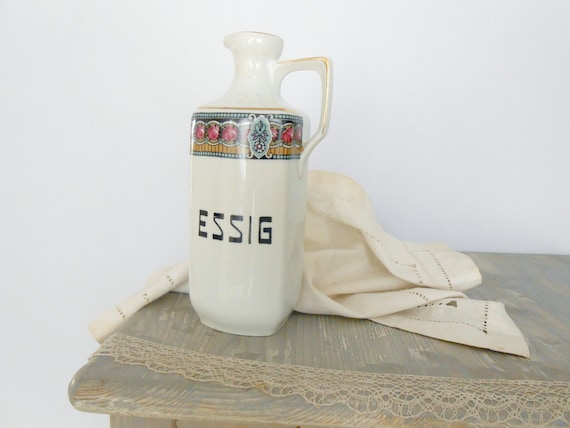This photograph features a vintage ceramic or glass pitcher prominently placed at the center. The pitcher is entirely white, accentuated with a gold streak along its handle and a gold band around the top. Adorning the upper part of the pitcher is a detailed border with a tribal-like pattern featuring hues of red, green, and mustard yellow, possibly with grape motifs, suggesting it may have been used for wine. The letters "E-S-S-I-G" are boldly inscribed in black near the bottom of the pitcher. The backdrop includes a light gray wall extending from the top through to the bottom left corner, enhancing the rustic aesthetic. The pitcher rests on an old, light gray-brown wooden table, which appears to have a whitewashed look. Draped behind the pitcher is a beige cloth or lace doily, and in front of the pitcher, a dull gold netting pattern subtly adds to the intricate setup.